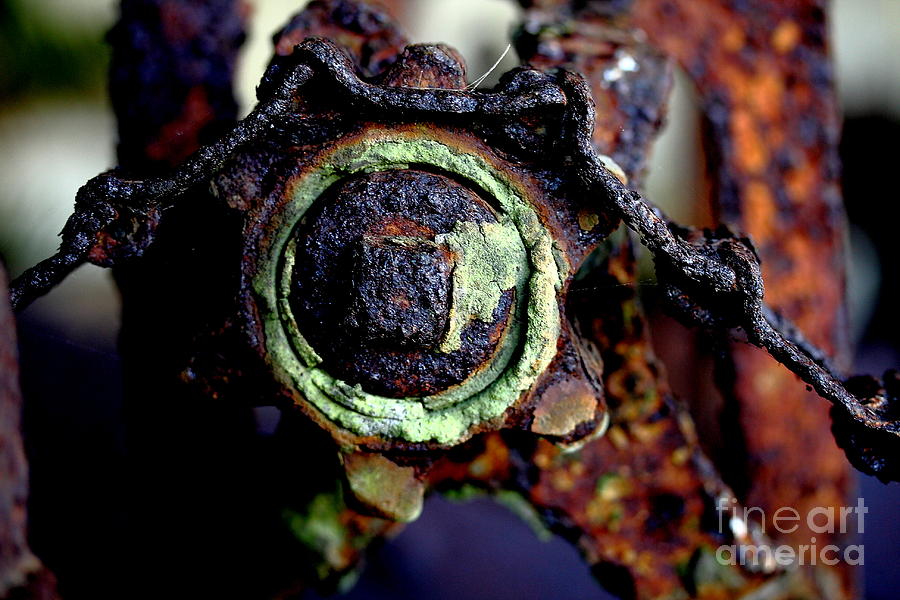This image, titled "Rusty Old Farm Equipment 7" by Wings Domain Art and Photography, captures a detailed up-close view of a corroded, cylindrical metal object. The central figure is heavily rusted, exhibiting various shades of brown and orange rust, with notable patches of bright green and yellow corrosion. The object is round with cog-like points and features a square bolt at its center, surrounded by a ring of green oxidization. There is a chain connected to the top, veering down to the left side, further adding to the sense of decay. The background is blurred, showcasing additional rusted metal pieces, suggesting more dilapidated equipment. The photograph is in landscape orientation, and the bottom right corner features a watermark that reads "Fine Art America" in white. The overall aesthetic is one of weathered industrial artistry, emphasizing the passage of time on metallic surfaces.